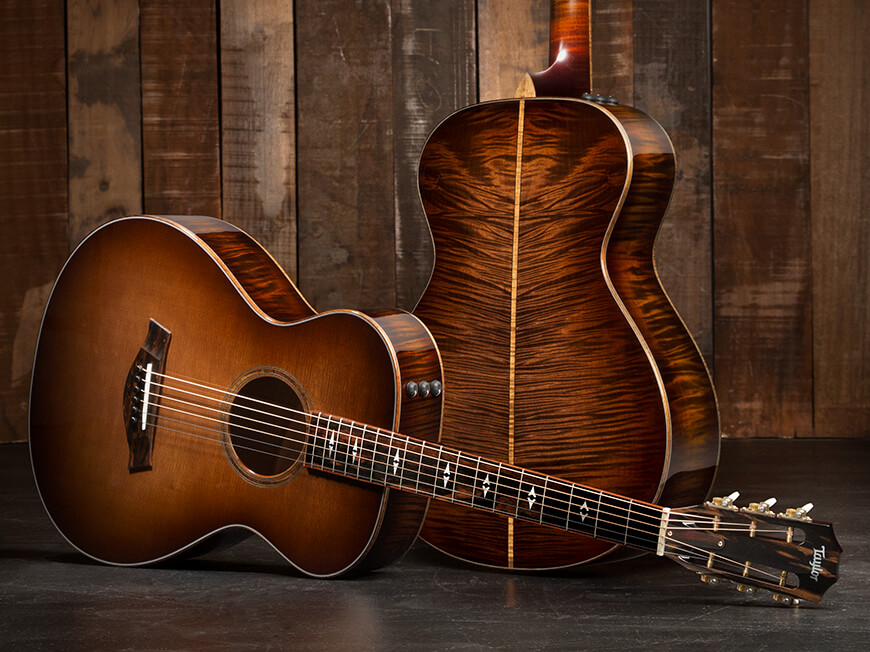This image showcases two acoustic guitars against a rustic vertical wooden plank wall. Both guitars exhibit a rich brown hue with the wood grain prominently visible, giving a shiny, polished appearance. One guitar lies on its side, revealing the front, which features a light brown center that darkens towards the edges. The neck of this guitar is a darker brown with white diamond-shaped inlays, and the headstock bears the name "Taylor" in pearl-like material. The second guitar stands upright, displaying its back, where a striking tiger stripe pattern of flamed maple is evident. A golden line runs down the middle of the back, adding to the intricate detailing. The floor beneath the guitars is black and gleaming, enhancing the overall contrast and highlighting the lustrous finish of the instruments.